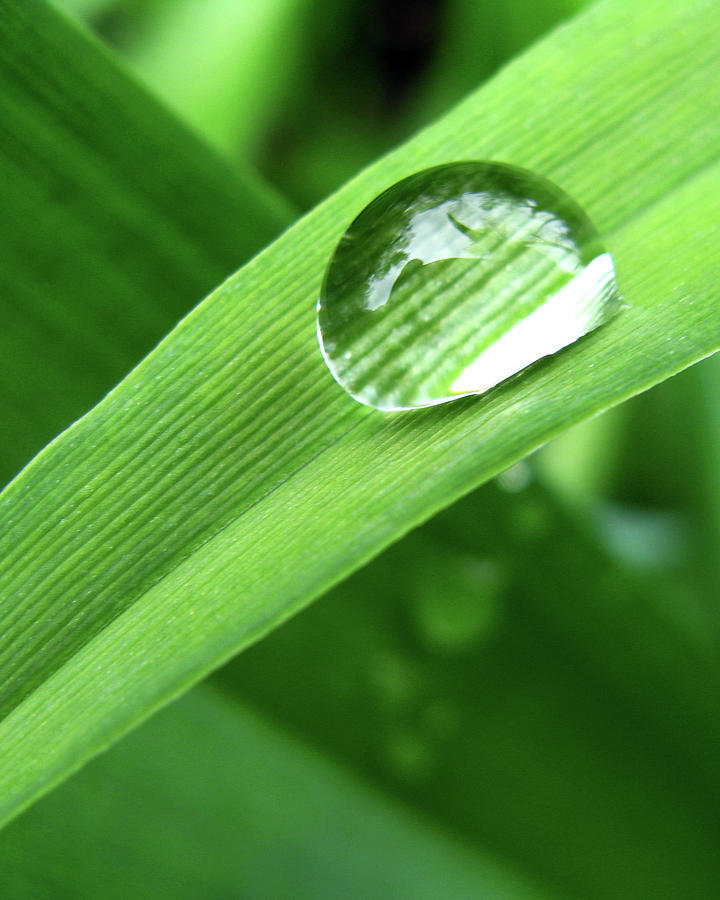This ultra-close-up image captures a single blade of grass in striking detail. The vibrant, healthy green of the blade is in sharp focus, revealing every fine striation. The center of the blade is adorned with a perfectly rounded droplet of water, acting like a tiny magnifying glass that enhances the intricate details of the grass beneath it. The droplet glistens due to the excellent lighting, and it reflects a hint of the sky above. Surrounding the sharply focused blade and droplet is a blurred green backdrop with hints of other leaves and additional water droplets, adding depth to the composition. The overall simplicity of the elements—a single blade of grass, the dew drop, and the green tones—creates a stunningly beautiful and serene image.